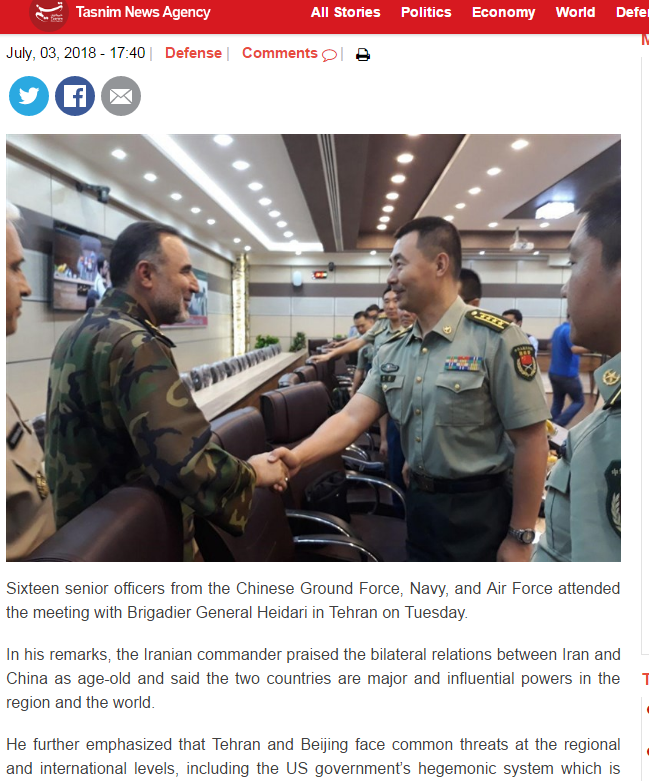This is a meticulously detailed cropped screenshot of the Tasnim News Agency website. The top of the image features a prominent red banner. On the top left corner, the label "Tasnim News Agency" is displayed accompanied by the agency's logo positioned just to its left. On the right side of the banner, there are navigation options labeled "All Stories," "Politics," "Economy," "World," and partially visible "D.E.F.E." likely indicating "Defense."

Beneath the red banner on the left side, the date "July 3rd, 2018," and the time "17:40" are visible under the category "Defense." To the right of "Defense," there's a section labeled "Comments," both displayed in red text, along with a page icon. Below these elements on the left, there are three round social media icons: Twitter, Facebook, and an envelope symbolizing email.

Dominating the upper part of the article section is a large photograph depicting two military men shaking hands, lending a strong visual emphasis. The article itself is partially visible below this image, but both the right side and bottom parts of the article are cropped out, leaving the full content obscured.